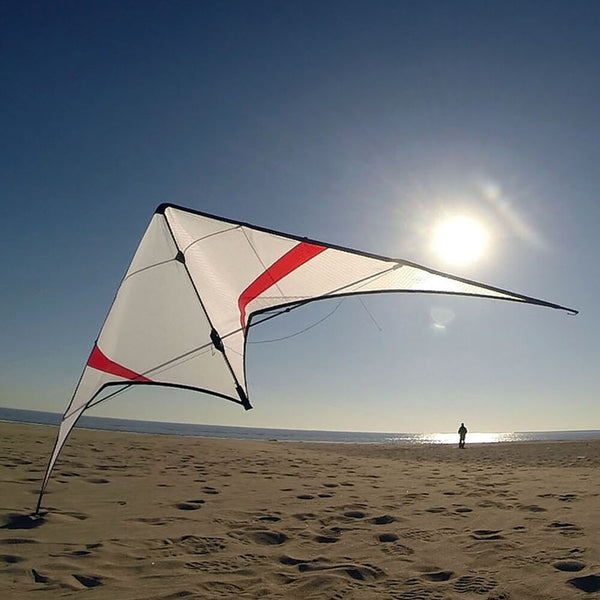A serene beach scene captured during twilight, with a sizable, intricate kite positioned prominently in the sand. The sky's ambiguous hues suggest either a sunrise or sunset, as the sun hangs low on the horizon. The beach is expansive, blanketed in sandy brown footprints and tracks, hinting at recent activity. The water in the background is calm, almost still, adding to the tranquil ambiance. Standing near the water's edge on the right side of the image is a person, possibly from the group managing the kite.

The kite itself is impressive in scale, with an aircraft-like triangular design. Its body is primarily white, accented by black trim and two distinct red lines on either side, adding a vibrant contrast. This kite is not airborne; rather, it is in a resting position with one of its corners embedded in the sand, creating an illusion of hovering with the other side slightly elevated. This placement indicates that the kite might either be preparing for flight or has just landed gracefully.